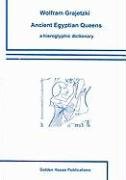The image appears to be a cover for a book titled "Ancient Egyptian Queens: A Hieroglyphic Dictionary" by an author likely named Wolfram Gragelital. The cover features a white background with dark blue-teal horizontal lines separating different sections of text and imagery. Central to the cover is a sketch that might depict a person, possibly holding flowers. The author's name is somewhat obscured and challenging to decipher. At the bottom of the cover, there is further text and potentially a publication logo, both of which are unreadable due to the poor image quality and small size. The overall design is simplistic, with text both above and below the central sketch, separated by distinct colored lines.